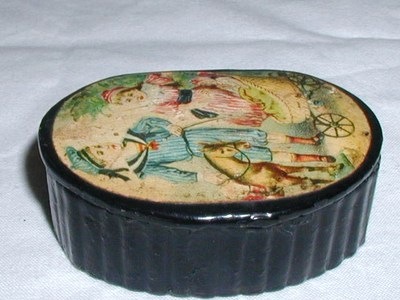The image depicts an antique ceramic object, possibly a casserole dish with a lid, photographed on a soft, slightly fuzzy gray-to-white background. The dish's sides feature scalloped edges reminiscent of a muffin, and it is a dark blue to dark gray color with a black ring around the top edge. The top surface of the lid showcases a painted scene that is not oriented in a straightforward manner in the image, with the top of the painting aligned to the left side.

The painted scene includes a young boy dressed in an old-time sailor outfit with blue and white vertical stripes, knickerbocker-type pants, and a sailor cap with ribbons hanging off the back. The boy, who appears to be under ten years old with short blonde hair, has a miniature horse positioned to his right that reaches just up to his hip. To the boy's left, there is a girl in a red or pink dress with a dark blue sash, along with a red ribbon or hat in her hair. In front of the girl, there is a small bassinet on wheels with a green blanket inside. The bassinet has three wheels, with the front wheel being black with several spokes and situated near the boy's left foot. Surrounding these figures is a backdrop that includes depictions of trees, contributing to the antique, old-fashioned charm of the scene.